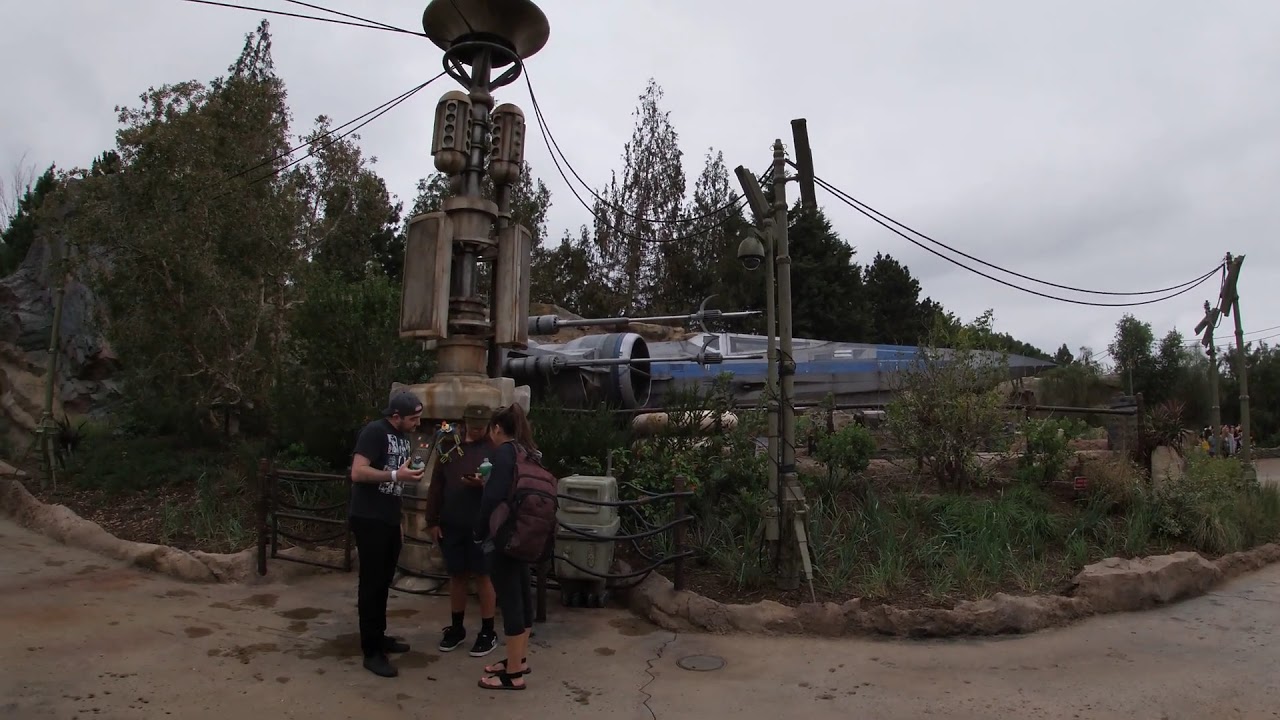In this outdoor scene, a striking blue and gray rocket is prominently displayed at the center, enclosed within a fenced area adorned with tall poles connected by wires. Three people stand in the foreground, conversing near the base of the rocket. Among them is a girl on the right, identifiable by her brown hair, maroon backpack, and black sandals. She is joined by two companions, one wearing black shoes, a gray hat, and a brown hoodie, and the other clad in a black shirt, black pants, and a backward cap. Behind them rises a brown electric tower with multiple lines extending from its top, framed by an abundance of trees. The setting suggests a museum or park, potentially with a Star Wars theme given the rocket's resemblance to a ship from the franchise. The ground appears to be a mix of cement and hardened earth with a surrounding berm, and a dirty sidewalk stretches along the path. Overhead, the sky is cloud-laden, casting a diffuse light across the scene.